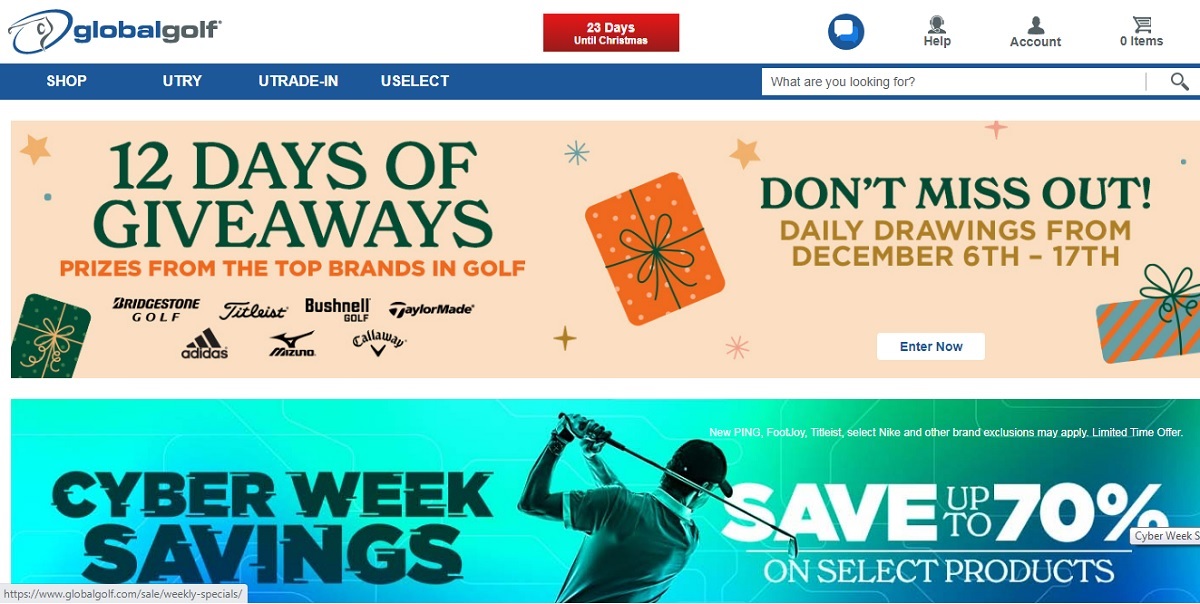In this promotional web page image, the word "Global Golf" prominently stands out at first glance, with "Global" colored in blue text and "Golf" in dark gray text. To the left of this text, there is a logo that depicts a person swinging a golf club.

At the top middle of the image, a box with a red background and white text announces "23 days until Christmas." The top right of the image features a small shopping cart icon, under which it states "0 items." To the left of the cart, the word "Account" is displayed, followed by "Help," and adjacent to these is a circular icon containing a white text box.

On the top left side of the image are navigation options such as "Shop," "You Try," "You Trade In," and "You Select," arranged horizontally, with an empty space in the middle. Further to the right, there is a search bar prompting "What are you looking for?" and at the far right end of the search bar is a magnifying glass icon, indicating search functionality.

Dominating the middle of the image is a festive announcement. On the left side, it reads: "12 Days of Giveaways, Prizes from the Top Brands in Golf." Central to the image is a graphic featuring an orange present. On the right, the text says, "Don't miss out, daily drawings from December 6th to the 17th." At the bottom right, a small green and orange present adds a final festive touch.